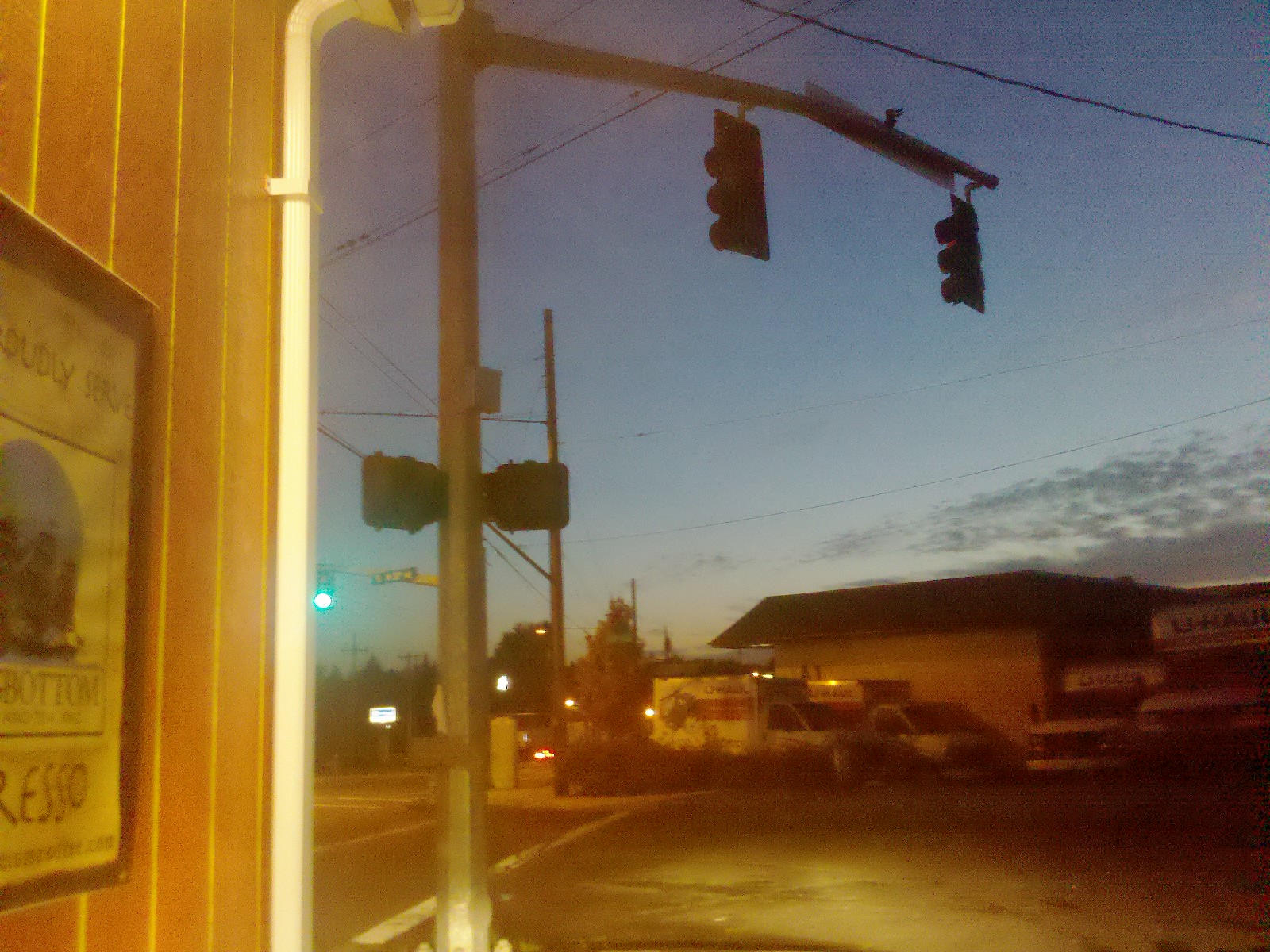A dark street corner captured just after sunset is illuminated by the soft glow of street lights, their reflections shimmering on the damp pavement. A few lingering clouds dot the twilight sky, adding depth to the scene. Dominating the right side of the image is a white-colored brick building with a dark, flat roof. In front of the building, two trucks, primarily white with striking red accents, are parked side by side. A traffic signal extends across the intersection, sporting two lights and a small caution light positioned lower on each side. On the left side of the image, a white wooden panel stands next to a reddish-yellow structure, both contributing to the urban aesthetic. A large sign hangs prominently on the side of the building, featuring red lettering and an illustrative graphic, completing this vivid depiction of a city street at dusk.